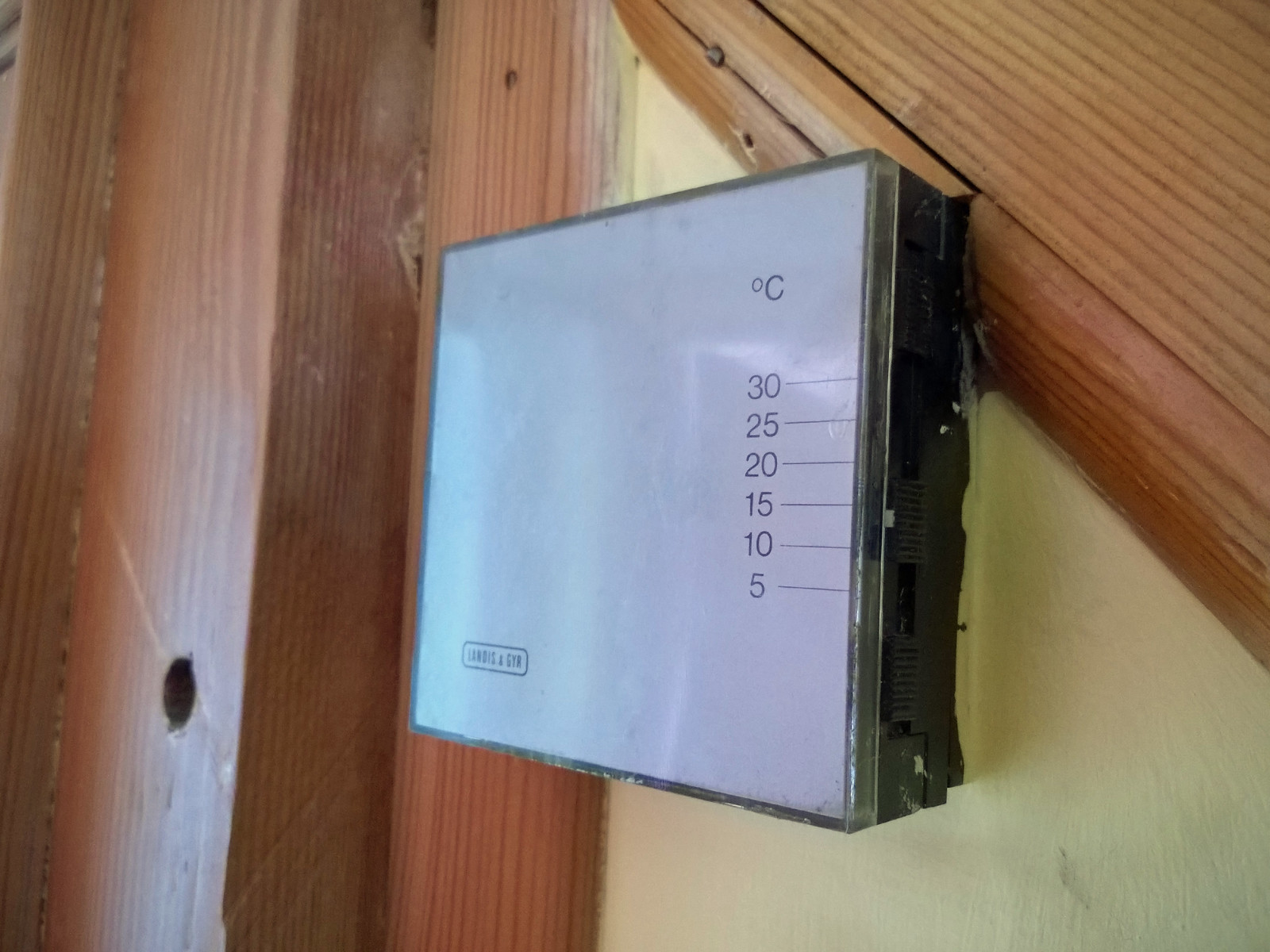The image depicts a television or digital screen mounted on a wooden wall with a yellowish-brown texture. The screen is roughly square-shaped with a black plastic frame surrounding a grayish-blue display. The screen itself seems to be covered in a plastic-like material, adding a slight gloss to its surface. 

The wall on which the screen is mounted features a horizontal-diagonal brown pillar above it, running from the top right to the bottom right. On the left side of the image, several vertical wooden pillars can be seen. The far-left pillar is particularly notable as it has a circular hole at its bottom-left corner and a large, visible scratch mark extending from the top left to the bottom right. Additional scratch marks are present towards the top-middle left side of this pillar.

On the screen, numerical values appear on the right side: 30, 25, 20, 15, 10, and 5, with the letter "C" above them. At the bottom left of the screen, a partially obscured name ending with "STR" is visible.